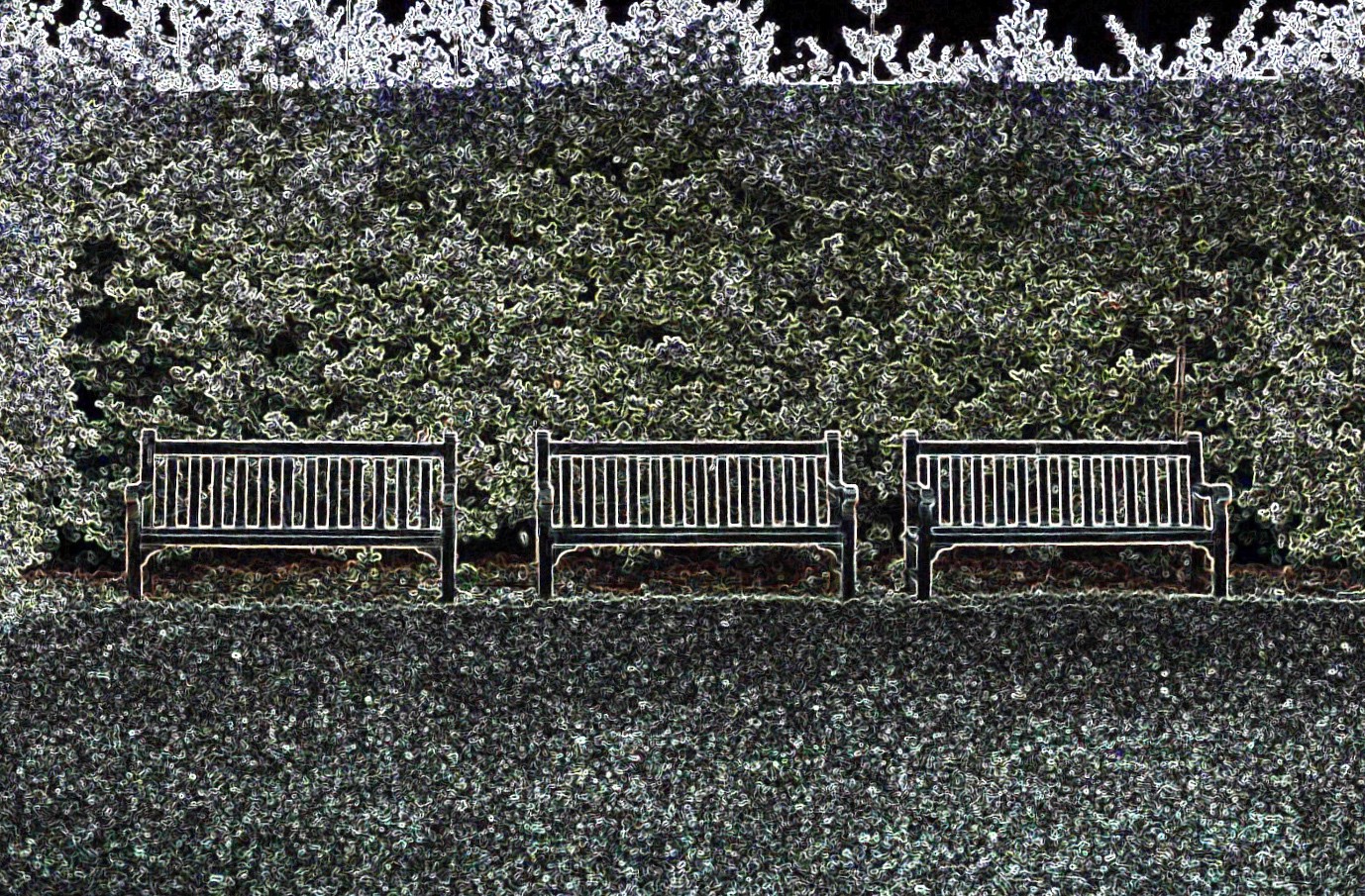This is an abstract, generated illustration resembling a photographic negative, showing three park benches set in a garden park area. The benches, appearing as hollowed-out shapes outlined in white, are arranged side by side on a dark lawn. A variety of hedges, vegetation, and trees form the background, with a mix of dark and light shades hinting at green. The sky, rendered in deep black, contrasts starkly with the white, intricate outlines of trees, bushes, and various flora behind the benches. The overall effect is a pixelated, high-contrast image with sporadic splashes of green and hints of purple and white, creating a surreal and somewhat eerie atmosphere.